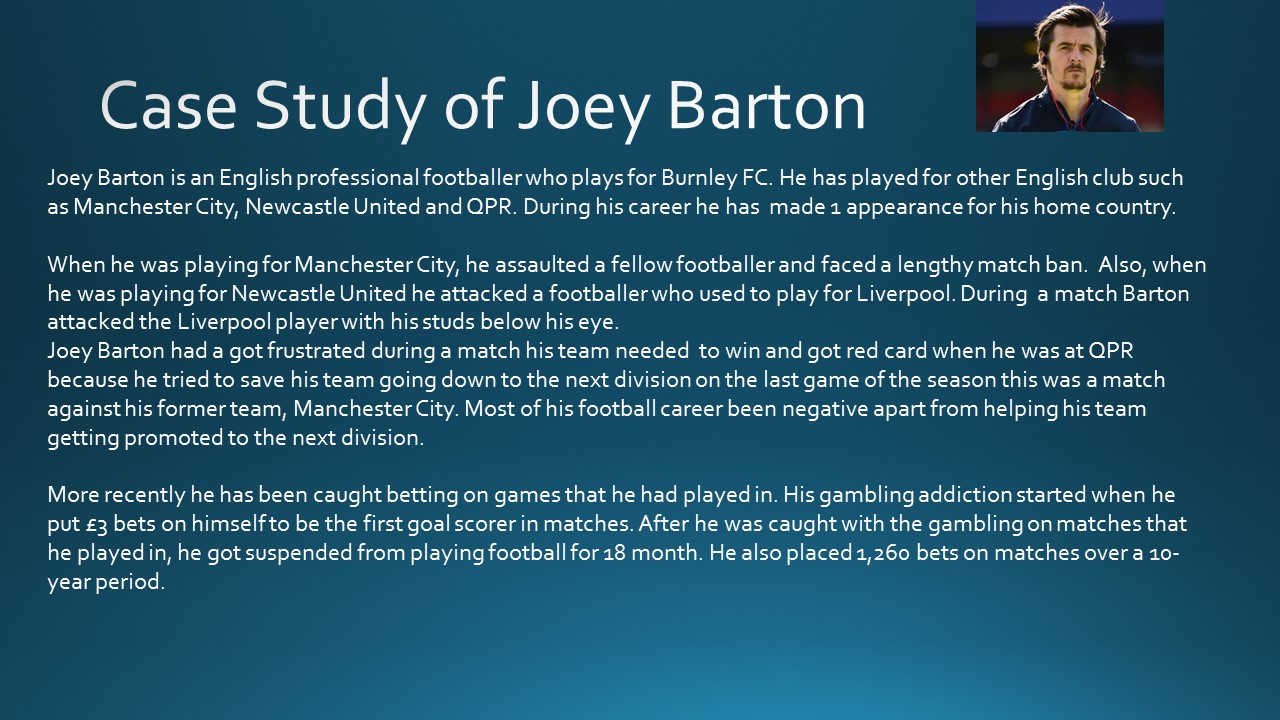The image depicts a slide from a presentation or possibly a webpage with a solid dark blue or greenish turquoise background. The central text, in white lettering, is titled "Case Study of Joey Barton". To the right, there is a photograph of Joey Barton from the shoulders up, showing a man with white skin, dark brown hair parted to the side, and a brown goatee. He is wearing a blue jacket and black headphones. The photograph is set against a brown and blue background. The text describes Joey Barton as an English professional footballer for Burnley FC, with a career that includes stints at Manchester City, Newcastle United, and QPR. It mentions that he has made one appearance for his home country. The text also discusses controversies, such as assaulting fellow footballers, betting on games he played in, and facing suspensions. The slide is formatted in a rectangular, horizontal shape with the text in three short paragraphs.